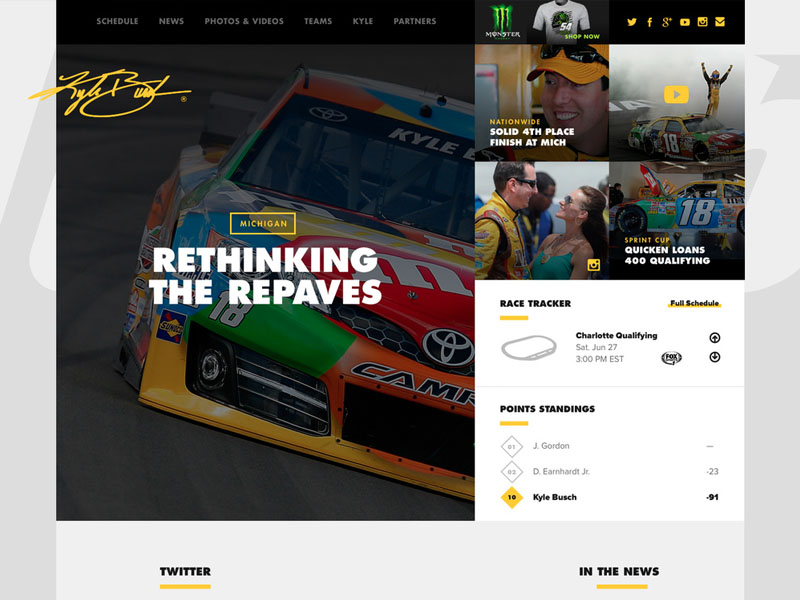The image depicts a detailed NASCAR-related website landing page. At the top left corner, there are six navigational categories displayed in gray text against a black background. These categories, listed from left to right, are: Schedule, News, Photos and Videos, Teams, Kyle, and Partners. 

To the right of these categories, the website features four square images showcasing various NASCAR themes. Above these images, a prominent Monster Energy logo is displayed as an advertisement. 

Moving further right, there are six yellow icons representing different social media platforms. On the left side of the page, there's an autograph in yellow located at the top left. Directly below it, within a yellow background or outlined yellow rectangle, the text "Michigan" is displayed. Beneath this, in white text, the phrase "Rethinking the Repaves" is written.

The central focus of the image is a front view of a NASCAR vehicle. The car features a mix of red, yellow, green, blue, orange, and black colors. The name "Kyle" is prominently visible at the top, indicating that it belongs to Kyle Busch, and the vehicle is identified as a Toyota Supra.

Below the image of the car, the word "Twitter" is written in black text with a yellow underline. At the bottom of the section, various headings are listed: Race Tracker, Full Schedule, Charlotte Qualifying (scheduled for Saturday, June 27th, at 3 p.m.), Points Standings. Kyle Busch is listed as the third option beneath Jay Gordon and Dale Earnhardt Jr.

On the far right, under an "In the News" section, the entire right-hand side of the image is set against a gray background.